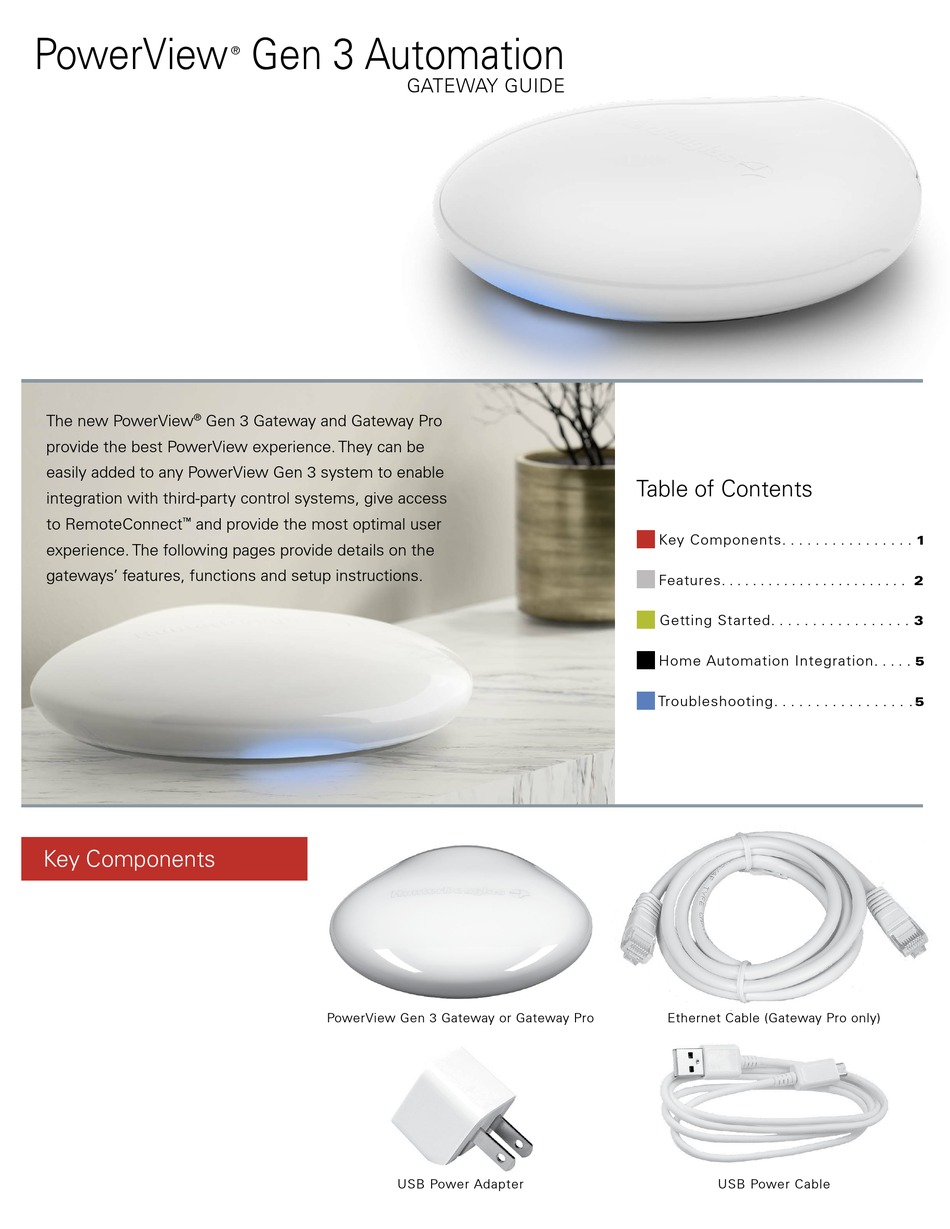Caption: 

The image showcases the "PowerView Gen 3 Animation Gateway Guide," featuring a sleek, white device. A blue line runs subtly in the background, adding a touch of modern elegance to the composition. The new PowerView Gen 3 Gateway Pro is highlighted as providing the best PowerView experience, seamlessly integrating with any PowerView Gen 3 system and third-party control systems. The guide promises comprehensive details on the gateway’s features, functions, and setup structure, referencing sections such as key components, features, game starter, home automation integration, and troubleshooting. Key components depicted in the image include the PowerView Gen 3 Gateway or Gateway Pro, the necessary cables, and the USB power adapter. Notably, the Gateway Pro features ports on both sides and a reflective surface to the right, contributing to its sophisticated design.